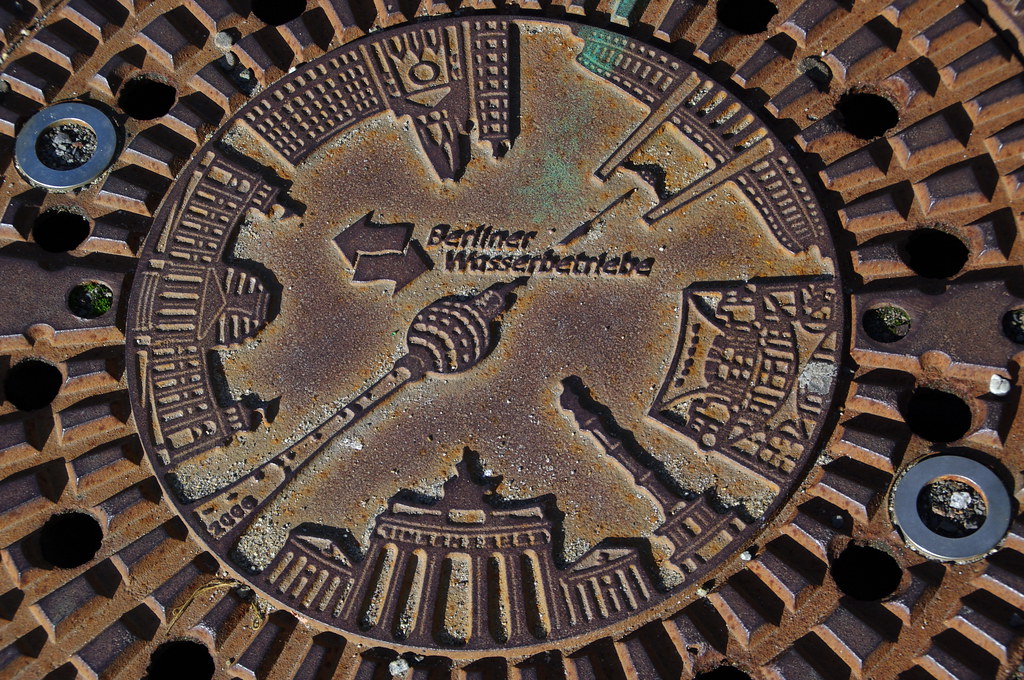The image depicts a rusted brown manhole cover with a rough, textured surface, possibly made from bronze or copper. The cover is circular with intricate designs etched into it, including various types of buildings like skyscrapers, government buildings with Roman columns, a Capitol-like structure, and extremely tall towers with spires. These buildings encircle a central text that reads "Berliner Wasserbetriebe," indicating a likely German origin. Surrounding the central design are broken lines and series of spaced black holes, giving it a grate-like appearance. Additionally, two partial silver rings are visible on opposite sides of the cover. The overall impression is that of a weathered, ornate manhole cover that blends utility with architectural artistry.